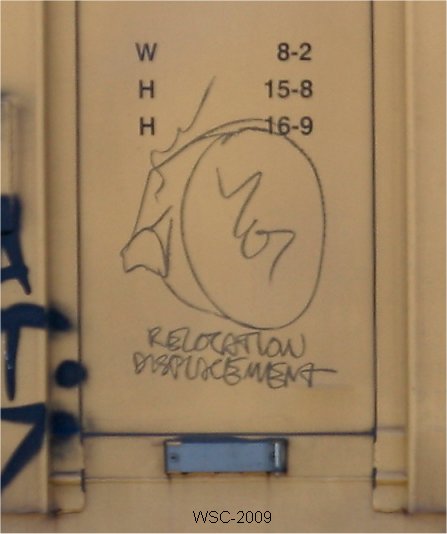The image captures a detailed view of a wall-mounted circuit box or metal wall plate against a yellowish or light brown background. Printed text on the wall plate includes "W82," "H158," and "H169" arranged in a column form. Handwritten in black graffiti are the words "relocation" and "displacement" in capital letters. Additionally, the graffiti includes "WSC-2009" at the bottom. There is black paint on the left side of the white background, complemented by a blue slot or blue spray paint along the edge. The setting provides a clear view of a silver metal strip central to the image, highlighting both the professional labeling and informal markings.